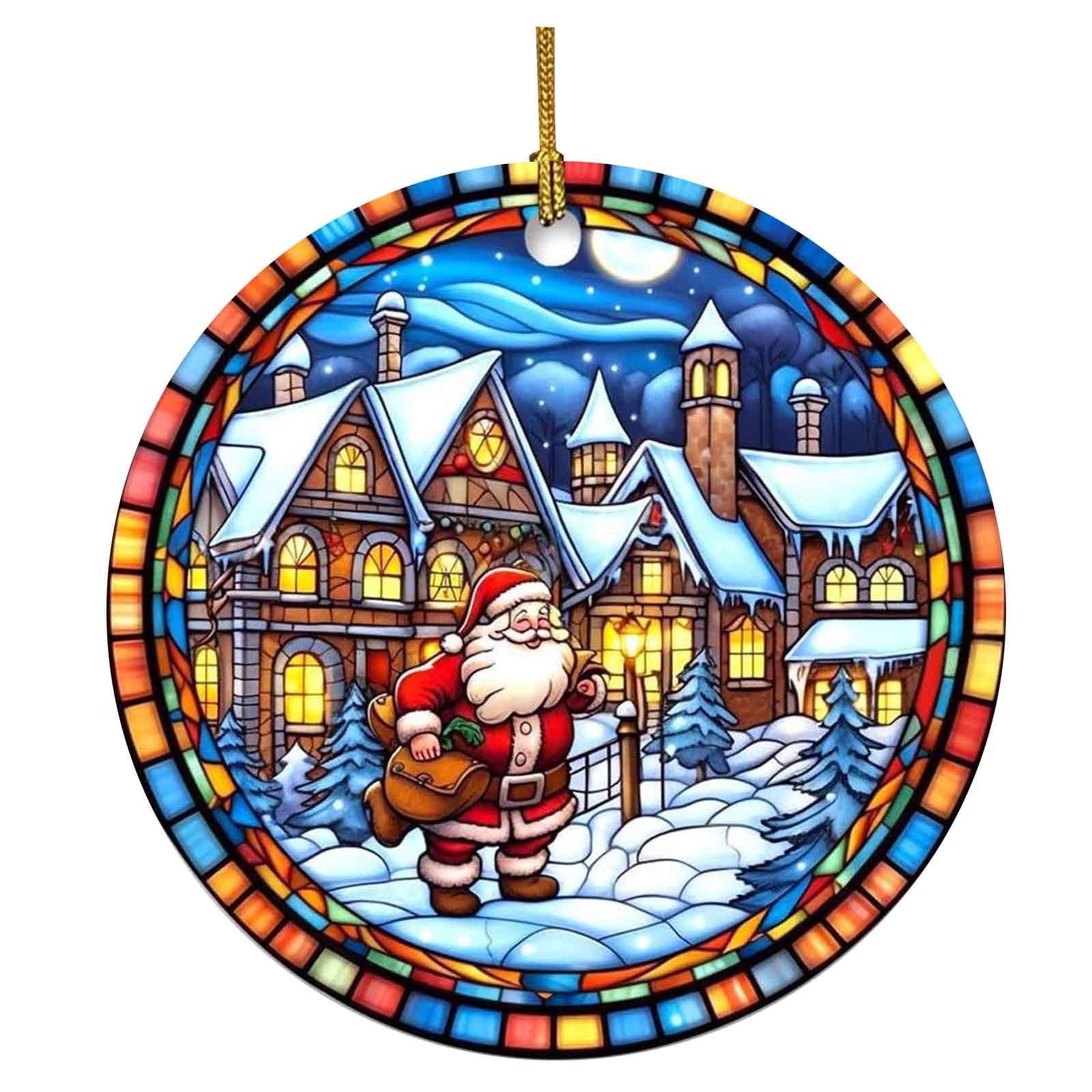The image depicts a computer-generated, circular stained-glass Christmas ornament, suspended by a braided gold thread. The ornament features a multicolored border composed of small rectangular and abstract stained-glass pieces in shades of red, blue, orange, yellow, and scattered green. At the center of the ornament, a cheerful Santa Claus stands on a snowy path, dressed in his traditional red jacket with white cuffs, white buttons, and a large brown belt with a silver clasp. He holds a light brown leather sack in his left hand. The background shows a quaint village with interconnected brick houses, their yellow-lit windows creating a warm glow through the stained-glass panel divisions. The rooftops are blanketed with snow, and a dark blue sky with a large blue-and-white moon overhead emphasizes the nighttime setting. Santa's rosy cheeks and the detailed colors, including reds, whites, browns, blues, and greens, add vibrancy to this festive depiction.